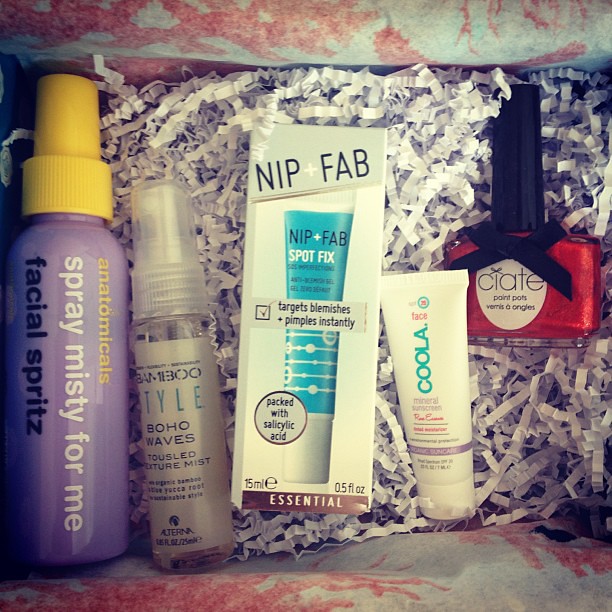The image displays an overhead view of a neatly arranged collection of beauty products nestled in white crinkled confetti within a decorative basket that has white and pink sides. On the left, there's a purple spray bottle with a yellow cap labeled "anatomicals spray misty for me facial spritz." Beside it, there's a smaller clear spray bottle labeled "bamboo style boho waves." In the center, a boxed product labeled "Nip + Fab Spot Fix" promises to target blemishes and pimples instantly, noting it is packed with salicylic acid and marked as essential. Next to this, a small tube of "Coola Mineral Sunscreen" is visible, and to the right, a bottle of red nail polish with a black lid and a black ribbon, labeled "Ciaté Paint Pots," completes the ensemble.